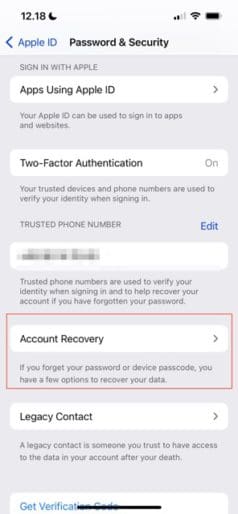A screenshot of an iPhone displays a security and privacy settings page, captured in portrait format. The status bar at the top shows the time "12:18" with a black moon icon indicating a nighttime theme. On the right side of the status bar, Wi-Fi signal and battery level icons are visible.

Below the status bar, the screen is divided into several sections. At the very top, a header says "Password and Security" in black text. To the left, a blue label reads "Apple ID," accompanied by a blue arrow pointing to the left, suggesting a navigational option.

The main content starts with a section titled "Sign in with Apple," containing a white box with the text, "Apps using Apple ID." Below that, it explains that, "Your Apple ID can be used to sign into apps and websites."

Further down, a section in white text announces, "Two-Factor Authentication: On," indicating that this security feature is enabled. It explains that trusted devices and phone numbers are used to verify identity during sign-ins.

The next part highlights "Trusted Phone Number" with a blue "Edit" button next to it. Beneath this is a mosaicked image and additional text explaining that trusted phone numbers are used to verify identity and assist in account recovery if the password is forgotten.

The subsequent section is bordered in red and titled "Account Recovery." It explains the options available for data recovery if the password or device passcode is forgotten.

The final section, "Legacy Contact," describes that a legacy contact is someone trusted to access account data after the user's death.